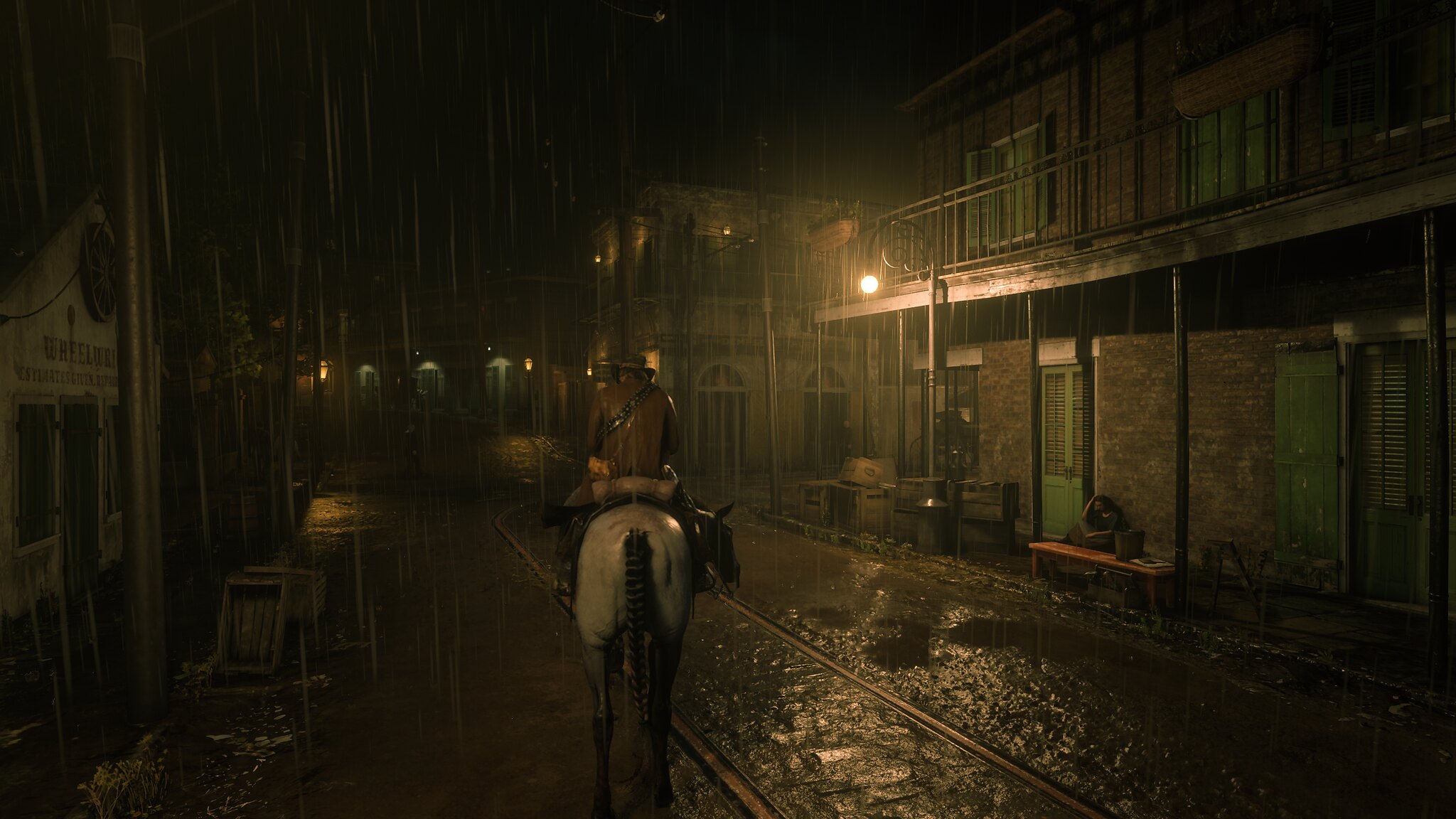In the nighttime rain, a scene unfolds that evokes the spirit of a Western town or perhaps the historic charm of New Orleans. The left side of the image features an ambiguous sign, partially visible to reveal the word "Wheel" followed by letters that might be "W," "R," or "A," obscured by the elements. Beneath this sign, indistinct words hint at something else written there, challenging interpretation in the dim light.

Dominating the composition is a statue capturing the back view of a figure clad in a cowboy hat and a brown jacket, with a satchel slung across his torso. The figure is astride a striking white and black horse, lending an air of rugged nostalgia to the scene. This entire tableau stands resilient under the pelting rain, adding a somber, almost poetic touch to the atmosphere.

Adjacent to this scene, nestled beneath a building of red brick with verdant green doors, a solitary figure sits huddled. Wrapped in a blanket, the figure suggests a life of hardship, possibly homeless, seeking refuge from the incessant rain. The image is a vivid juxtaposition of monumental stoicism and human vulnerability, illuminated softly by the reflections from the wet surfaces around.